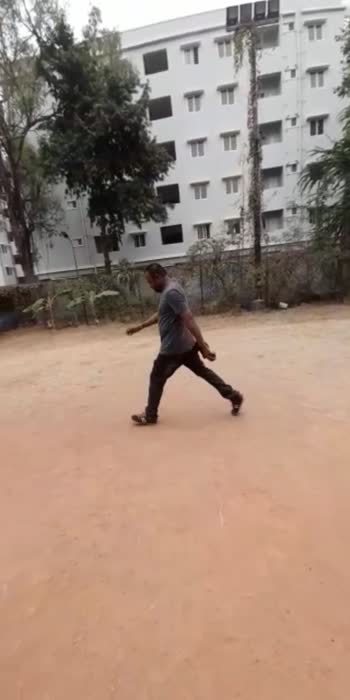In this photograph, the central focus is a man walking through a large, barren dirt field. He is positioned directly in the middle of the image, taking long strides with one foot forward and the other back. Wearing a gray t-shirt, dark pants, and sneakers, he walks purposefully towards the left side of the frame. The image is slightly tilted downwards to the left.

Behind the man, a chain-link fence separates him from a backdrop of unkempt weeds, shrubs, and three tall trees. Climbers and plants partially obscure the fence. Further behind, a towering white building with multiple stories and numerous windows rises against a pale sky that is nearly indistinguishable due to the bright daylight. The environment and overall setting suggest that this could be in a third-world country, possibly in an urban area behind a building or in an undeveloped lot.